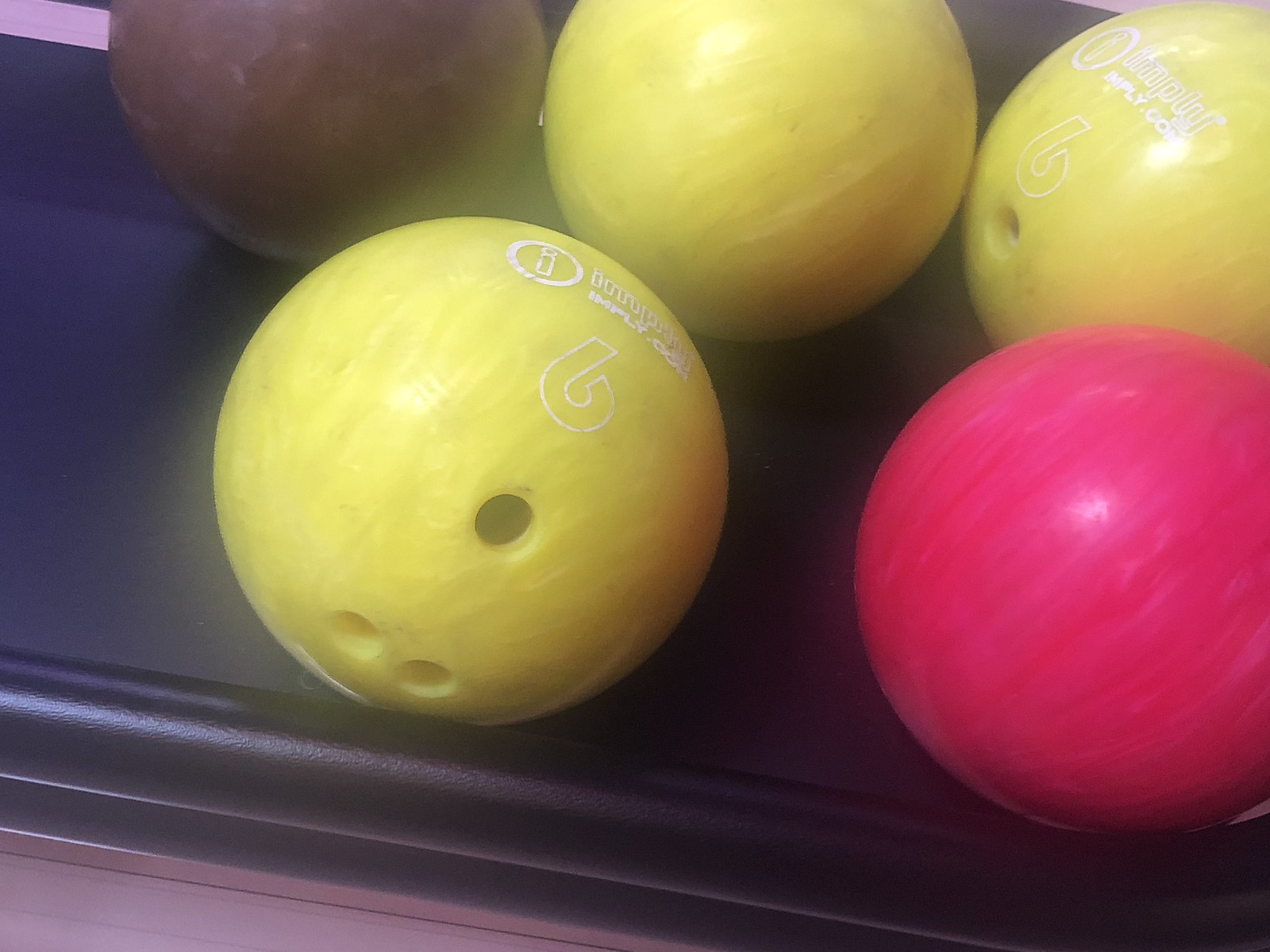The image depicts a set of five bowling balls situated on a black return tray with a rubber edge, likely at a bowling alley. The background showcases a blend of pink and purple hues. The bowling balls are arranged with three on the top row and two on the bottom. The top row features a brown ball on the left and two yellow balls to the right, with one showing three finger holes and the other one hole. On the bottom row, there is a yellow ball with visible white writing and three holes, placed on the left, and a pinkish magenta ball on the right, which appears solid without any visible holes. Faint glimpses of a brown wood floor are noticeable in the top left and bottom left corners of the image. The yellow balls feature a white swirl pattern, contributing to a sense of cohesion and design uniformity.